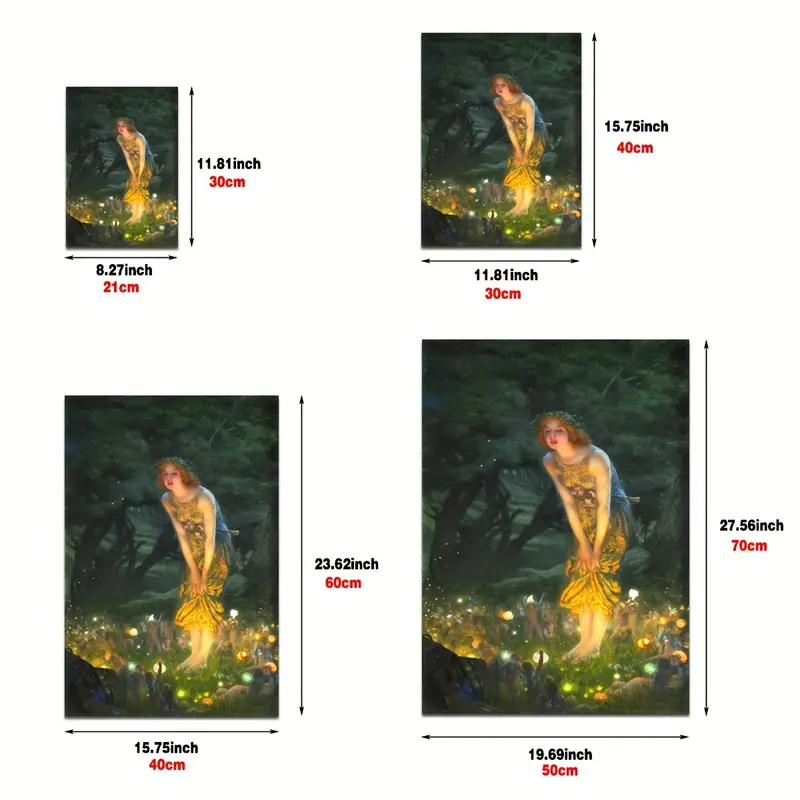The graphic consists of four identical images displayed in varying sizes against a white background, likely for the purpose of showcasing available print sizes for purchase. The image, a famous yet unnamed work of art, depicts a young woman with shoulder-length reddish-brown hair and very pale skin standing in a nighttime forest. She's wearing a flowing yellow and green dress and is barefoot, slightly pulling up the bottom of her dress near her knees. The woman is adorned with a wreath of flowers on her head and is leaning forward, seemingly admiring the tiny fairies and their glowing lights that illuminate the grass at her feet. The scene is enriched by darker, ominous clouds and the presence of a dead tree. The artwork is shown in four different sizes: 21 by 30 centimeters, 30 by 40 centimeters, 40 by 60 centimeters, and 50 by 70 centimeters, positioned clockwise from the top left corner. The smallest dimension in the top left is noted with additional measurements: 8.27 inches across the bottom and 11.81 inches from top to bottom. This detailed layout suggests a catalog or web display to guide potential buyers in selecting the desired print size for their homes.